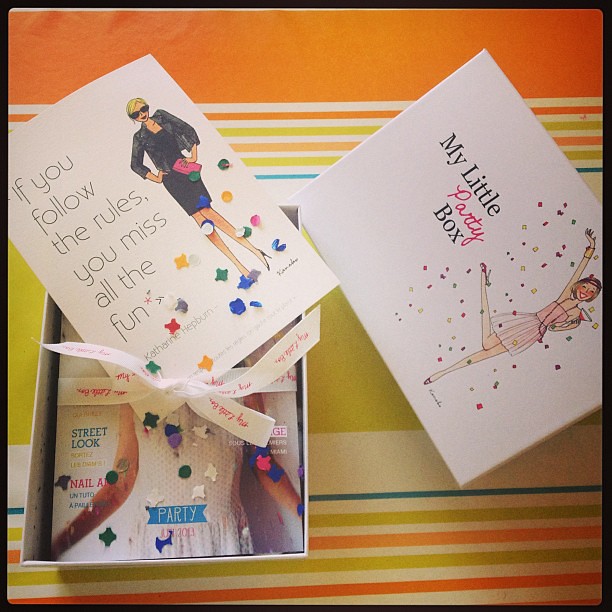The image depicts an opened sampler box placed on a colorful, striped placemat featuring shades of orange, white, green, and blue. The box’s lid, positioned to the right side, prominently displays the title "My Little Party Box" alongside a whimsical drawing of a light-skinned woman dressed in a strapless pink dress. With her knee slightly bent, she joyfully holds up a wine glass filled with a red drink amidst a shower of multicolored confetti. Inside the box, some items are neatly bound with a pink ribbon, and atop them lies a flyer. This prominent flyer, surrounded by confetti, bears the message "If you follow the rules, you miss all the fun," accompanied by a drawing of a woman with blonde, short hair, donning black sunglasses, a black jacket, and a matching skirt. The entire scene is set against a festive and vibrant backdrop that emphasizes the celebratory theme of the sampler box.